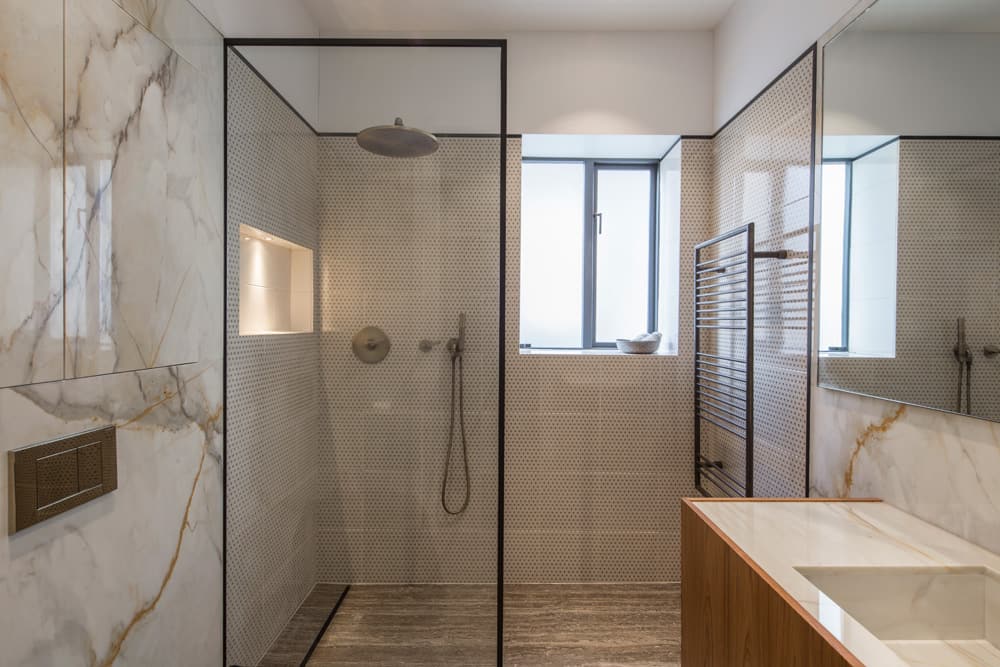The interior of the modern bathroom is a showcase of stylish simplicity and functionality. To the left, a marble wall, composed of light-colored panels with intricate black and orange veining, features a sleek, flat silver shower head with numerous tiny holes. Below this, a countertop of matching marble with a surrounding wooden frame houses a rectangular sink, topped by a mirror. 

In the heart of the space, the open shower concept stands out, with one glass barrier framed in black trim. The shower area, without a door, also features a frosted glass window allowing ambient light to filter through while ensuring privacy; a simple bowl sits on its sill. The shower boasts both an overhead circular shower head and a handheld shower device on a metallic hose, all controlled by a set of silver handles. A carved niche in the wall, illuminated by recessed warm lighting, provides storage for shampoo bottles, while a dark iron rack opposite offers a place to hang towels or laundry. The shower floor is made of brown concrete, accented by a textured tile design. The overall color scheme is dominated by cream, with contrasting black and yellow marbling, enhancing the contemporary aesthetic.